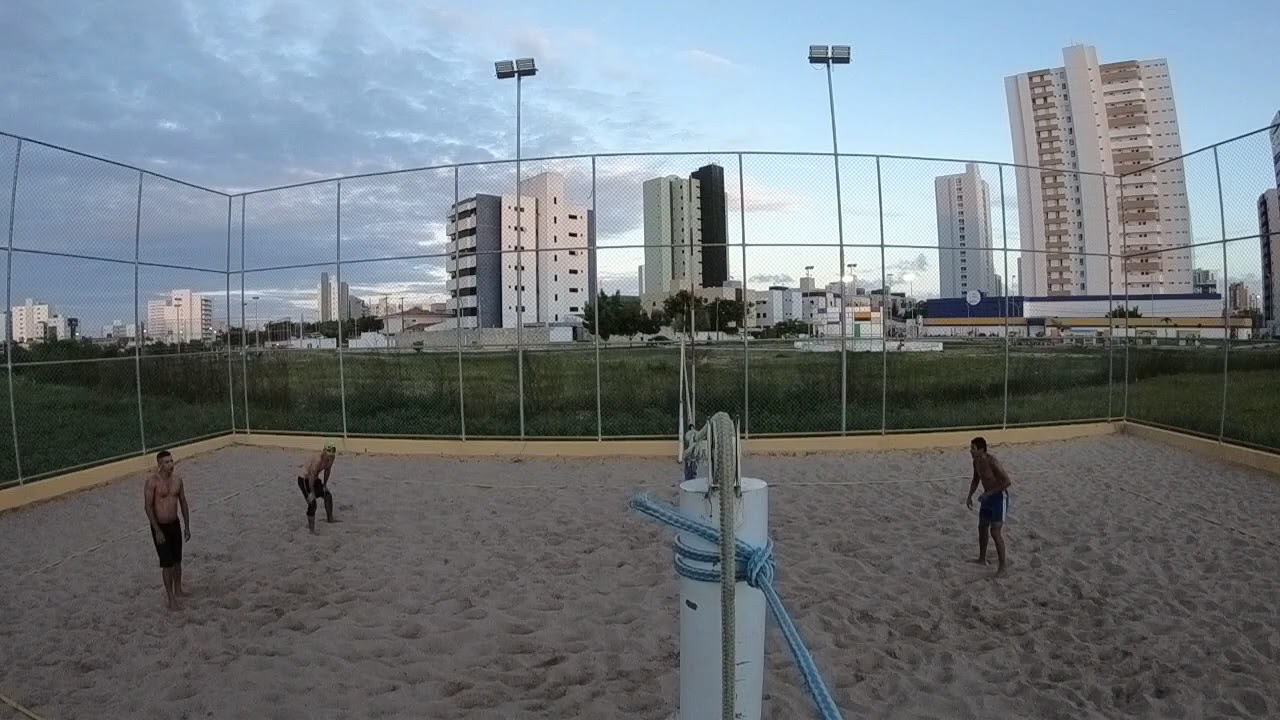The image captures an outdoor beach volleyball match set in an urban environment. The court, filled with light tan sand, is framed by a wooden or stone base and enclosed by a high chain-link fence with lights atop. Centered in the image, a white metal pole holds up the volleyball net. On the court, three topless men in swim trunks are ready for play - two on the left and one on the right. Beyond the fence lies a stretch of green grass and fields leading to a cityscape with various high-rises. The tallest building, a white structure, stands prominently in the upper right corner, with another smaller white building nearby. A blue sky filled with clouds crowns the scene, highlighting the harmony between the athletic activity and its urban surroundings.